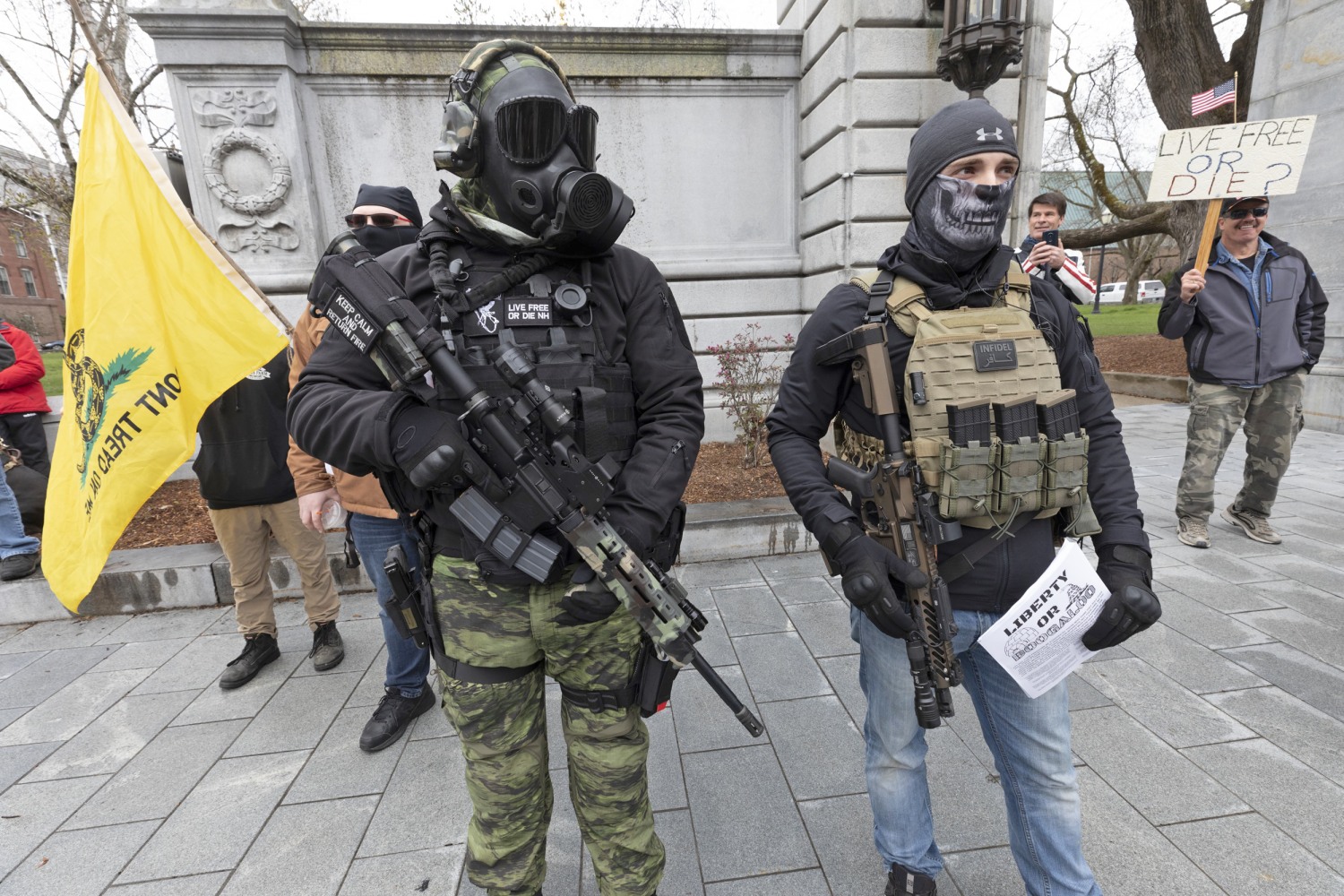The image depicts a protest scene with the primary focus on two individuals dressed in military-style gear. Both men are standing side by side, exuding a formidable presence. The man on the left is dressed in a black top and a bulletproof vest, paired with green camouflage pants. He is also wearing a gas mask and holding an automatic rifle. His counterpart on the right is equally imposing, sporting a gray Under Armour-style hat and a skull-patterned scarf covering his face. He has a gun slung over his right shoulder and is also equipped with a bulletproof vest. The intense atmosphere is further amplified by their tactical attire, indicating a high level of preparedness amidst the protest crowd.